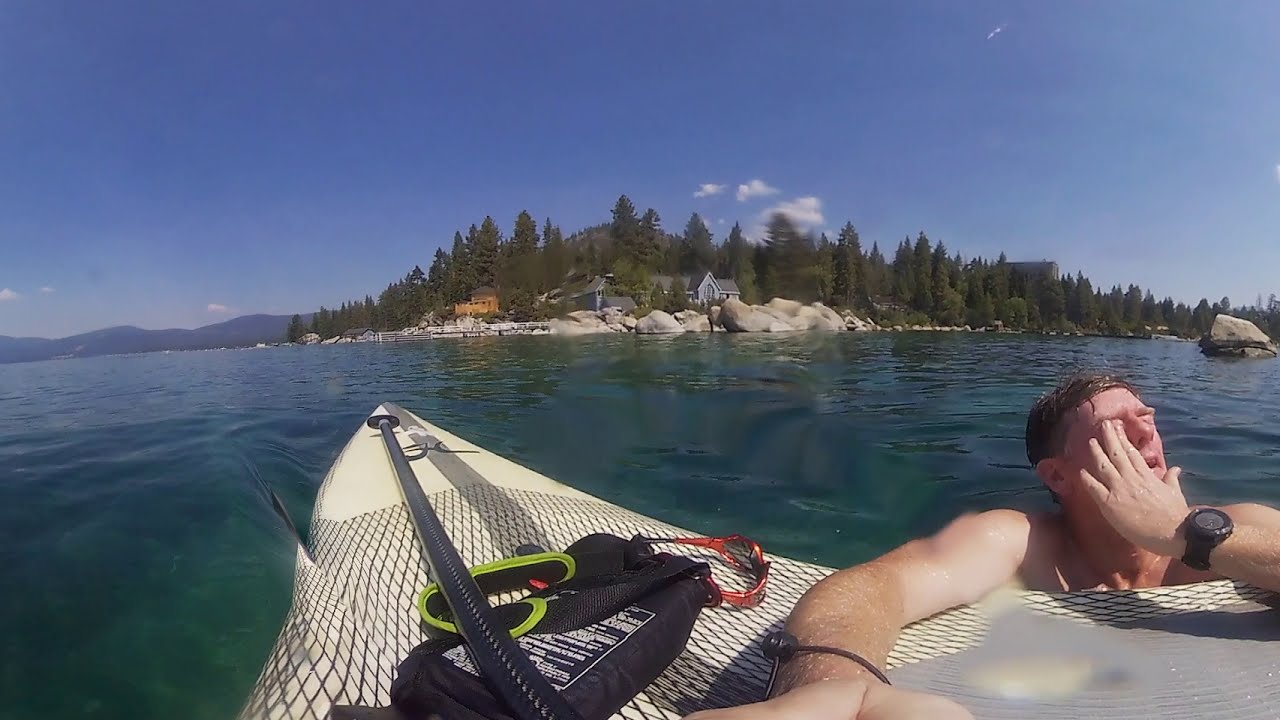In this detailed photograph taken from the perspective of a paddleboard on a lake, a man with a fair complexion is positioned on the right side of the image, partially immersed in dark blue water. He appears to be in the process of getting back onto his white paddleboard, which features a gray stripe running down the middle. With his left hand, which sports a black watch, he rubs his eyes, his copper-colored sunglasses perched nearby on the board. The board also holds a black and green life preserver and a black paddle. Surrounding this scene, the lower half of the image is filled with the rippling water, while the upper half opens up to reveal a shore lined with gray rocks, two houses painted in blue and brown hues, and a backdrop of vibrant green trees. In the distance, a majestic mountain range can be seen on the left side, beneath a partly cloudy sky filled with patches of light blue. The photograph captures a serene and detailed moment in nature, emphasizing the blend of outdoor adventure and scenic beauty.